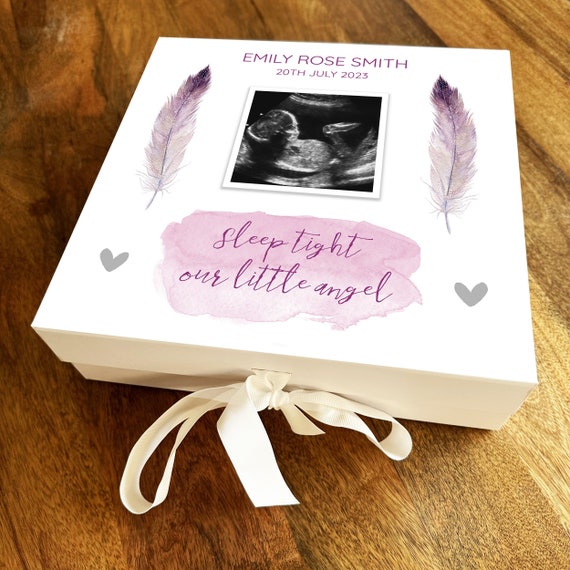This is a detailed photograph depicting a memorial keepsake box placed on a brown wooden surface. The box is predominantly white, though some descriptions suggest a light pink hue, and is adorned with a tightly tied ribbon at the front. Prominently displayed on the lid are the words "Emily Rose Smith, 20th July, 2023," indicating the significant event date.

Central to the box's design is a sonogram image, symbolizing a cherished memory. This image is flanked by two delicate feathers that exhibit a gradient of purplish-gray. Beneath the sonogram, in cursive script, the heartfelt message "Sleep tight, our little angel" is written, accentuated by a soft watercolor purple background. Additionally, two gray or silver hearts border this touching note.

The entire presentation suggests this box is a memorial tribute, likely commemorating a baby named Emily Rose Smith. The careful arrangement and gentle color palette convey a somber yet loving remembrance, with every detail — from the ribbon to the sonogram — thoughtfully placed to honor the memory encapsulated within.